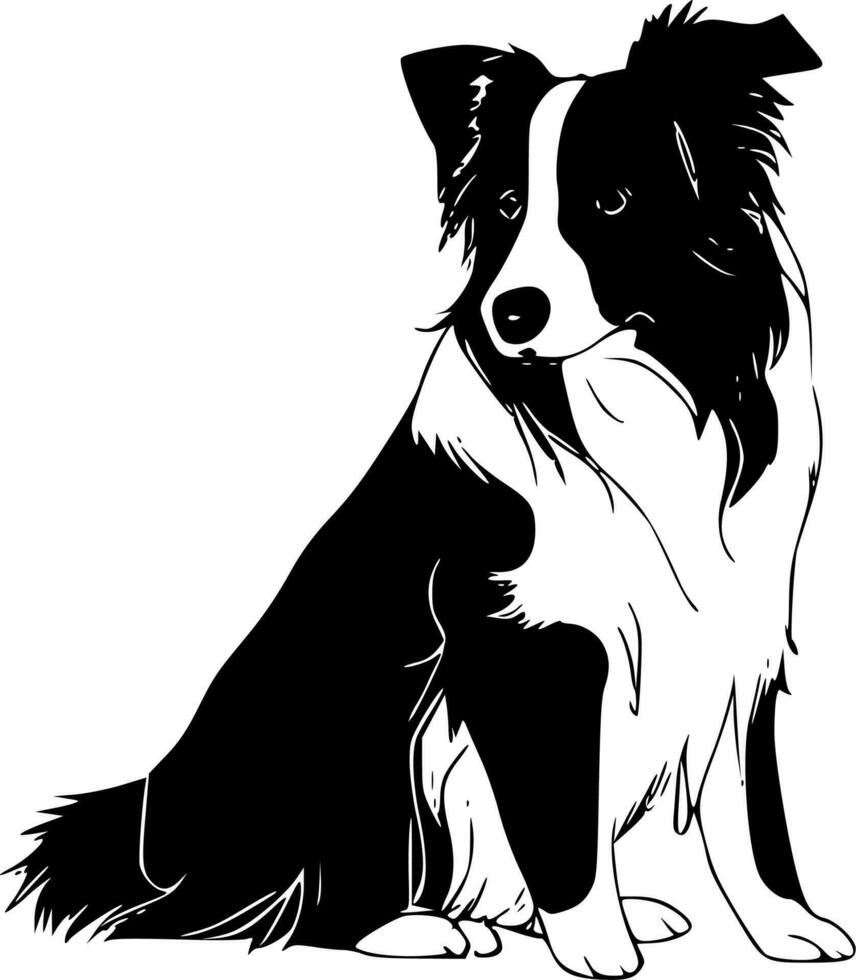This detailed black-and-white illustration features a potentially border collie dog, characterized by its long fur and alert posture. The dog sits with its hindquarters on the ground, facing to the left, with one ear drooping and the other raised as if something has caught its attention. Its body displays a striking contrast with predominantly black fur and a significant white patch on its chest and belly. The dog's face is defined by a white stripe running from its nose up across its forehead, which also matches the white fur on its muzzle. Its eyes, black like its nose, are wide open and attentively focused. This illustration is meticulously drawn, likely computer-generated, capturing a realistic, albeit not photographic, representation of the dog's charming and curious nature. The background is empty, devoid of any text or additional details.